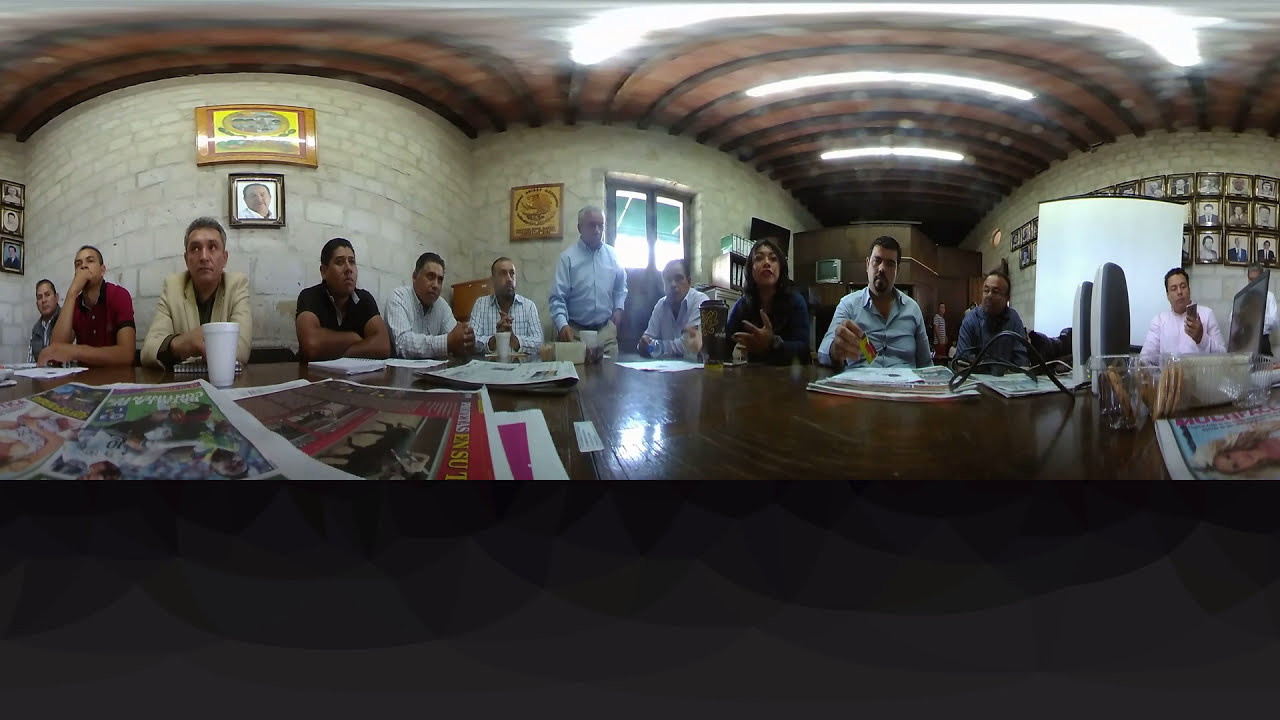The image depicts an indoor office setting where a group of people is engaged in a meeting or discussion around a large, dark wood table scattered with magazines, newspapers, coffee mugs, and biscuits. The room's walls are constructed of large white and tan-colored bricks held together by mortar. On the right wall, multiple portraits of people are meticulously arranged in rows. The left wall features a solitary photograph beneath a painting. The ceiling above exhibits an intricate design of light-colored wood with intersecting dark beams and fluorescent lights. 

Against the center wall, there is a doorway flanked by two large windows and adorned with a photo frame. The image shows a total of 12 people, with 11 seated and one standing prominently at the center of the table. Specific details include individuals on the left focusing forward, a woman speaking, and another person checking a mobile device in the far corner. Additionally, small speakers, files, and a TV are visible in the background, contributing to the busy, collaborative atmosphere of the room. Overall, the composition of the photograph suggests that it is a stitched panorama providing a comprehensive view of the attendees from multiple angles.